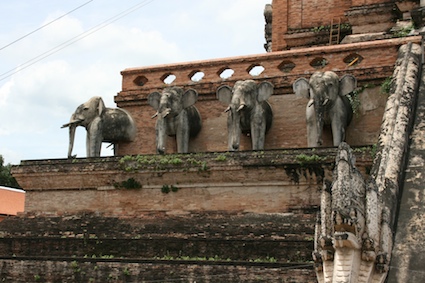The image depicts an ancient, weathered structure, possibly an old temple or ruin, adorned with four decorative gray elephant sculptures. These sculptures, embedded into the reddish-brown embankment of the structure, present only the front halves of the elephants, including their heads, two front legs, and tusks. The temple-like ruin comprises multiple layers: the bottom layer appears black with faded dark brown wood, the middle layer is light brown transitioning to regular brown with green moss, and the top layer is brown with circular cutouts, adding to the antiquated charm. To the right of the elephants, there is a indistinct, weathered white image and a small ladder. The background features a light blue sky with drifting white clouds and two telephone wires, enhancing the serene and historical ambiance of the scene.